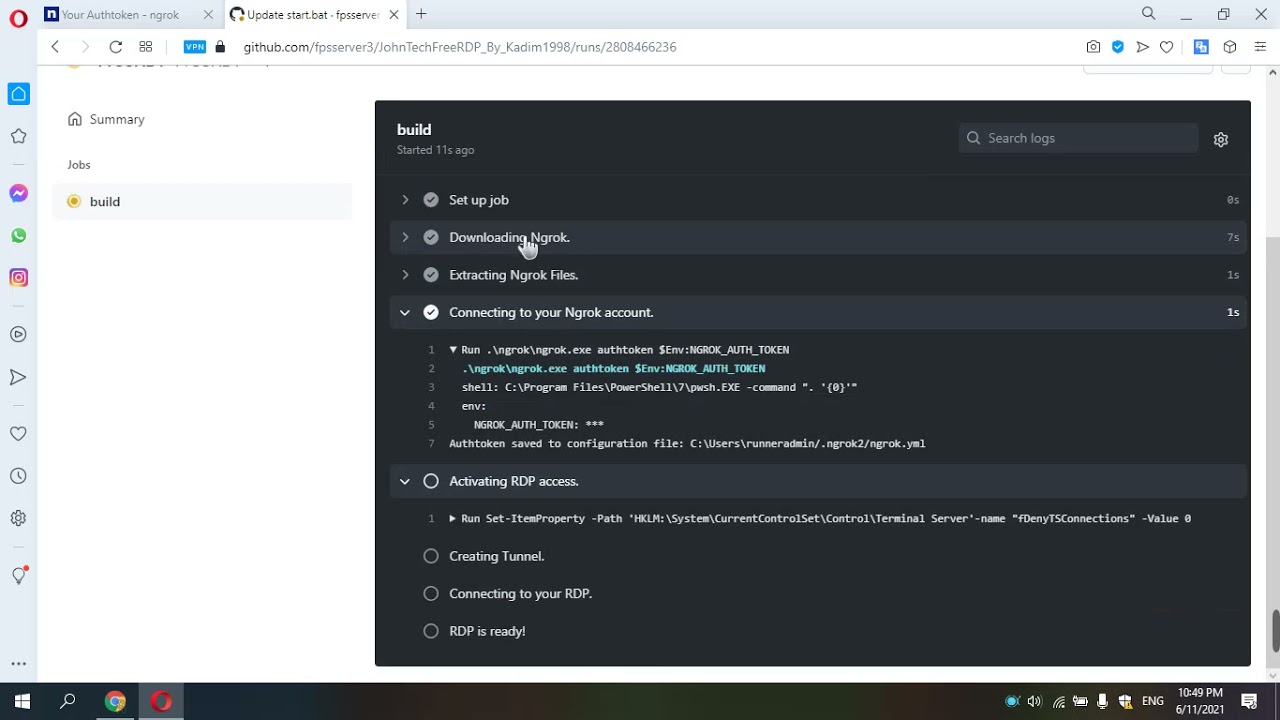A detailed and descriptive caption for the provided image could be:

---

The image appears to be a screenshot of a computer screen primarily showcasing an NGROK setup in progress on a web-based interface. At the very top of the screen, there's a characteristic NGROK logo—a stylized "N"—next to an authentication token field labeled "NGROK."

On the browser's tab bar, several tabs are visible. The active tab reads, "updatestart.bat.fpsserver..." but the rest of the title is truncated. A red circle indicative of the Opera browser is visible at the far left, suggesting that the Opera browser is in use.

The main part of the screen displays a GitHub page with the URL, "github.com/fpsserver3/johntechfreerdp_by_kadeem1988/runs/2808466236." This page is segmented into sections labeled "Summary," "Jobs," and "Build," with "Build" highlighted in light blue. It features a circular icon with an orange ring and center.

Directly to the right in a large, dark-themed console output area, the build process is documented. It starts with "Build started 11 seconds ago," followed by steps like "Setup job," "Downloading NGROK," and "Extracting NGROK files." Each completed step is marked with a gray circle containing a black tick, while the current task ("Connecting your NGROK account") is highlighted with a white circle and black tick.

The build process display lists further tasks such as "Run NGROK," detailing commands like "NGROK.exe auth token." Subsequent tasks include "Activating RDP access," “Run set item property path,” "Creating tunnel," and "Connecting to your RDP," although these steps have empty circles indicating they've yet to be reached.

At the bottom of the screen, the typical Windows operating system taskbar is visible, showing the time (10:49 p.m.), date (06/11/2021), and a series of icons including the familiar Windows symbol, an hourglass, shortcuts for Google Chrome and Opera, and system icons for sound, battery power, Wi-Fi signal, and security.

---

This edited caption provides a clear, detailed description of the image, emphasizing the visual and textual content present on the screen.